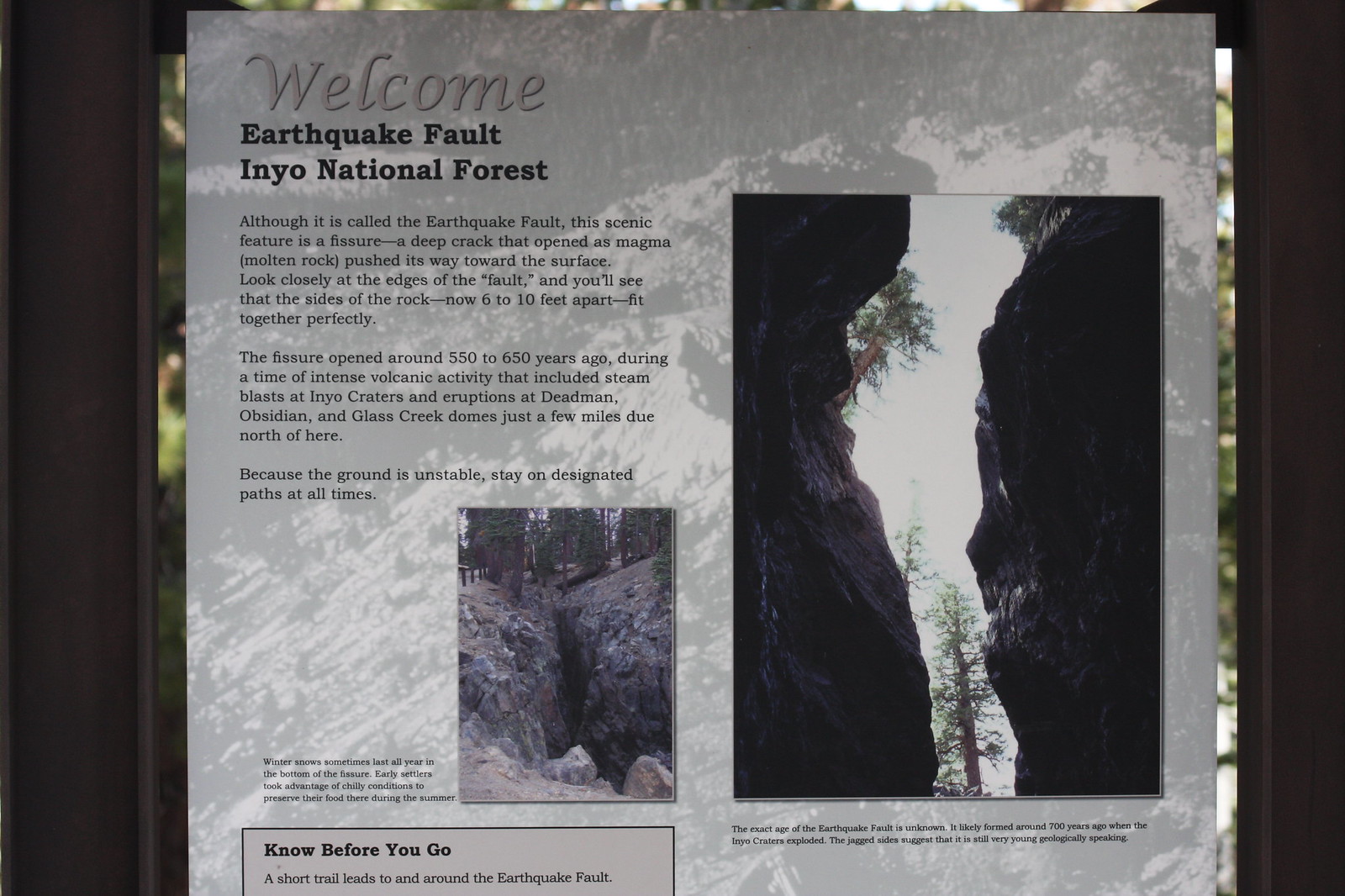In this black-and-white close-up image of a sign, we see a detailed description and imagery related to the Earthquake Fault in Inyo National Forest. The sign prominently displays "Welcome" in yellow text at the top left, followed by "Earthquake Fault" and "Inyo National Forest" in black text. Accompanying the text are two photos on the sign: one showing a scenic view of the forest with trees and another depicting a deep fissure between cliffs, likely emphasizing the Earthquake Fault itself. A comprehensive paragraph explains that the Earthquake Fault is actually a fissure, a deep crack created by magma pushing its way toward the surface. The text urges viewers to look closely at the edges of the fault, noting that the rock sides, now 6-10 feet apart, fit together perfectly. Additional information provided, though not fully readable, includes a "Know Before You Go" section that discusses the history of the fault, highlighting its formation around 550-650 years ago during a period of intense volcanic activity, and advising visitors to stay on designated paths for safety. The fissure, surrounded by cliffs and trees, also served early settlers as a natural refrigerator for food preservation due to the chilling conditions at its bottom, where winter snow can persist year-round.